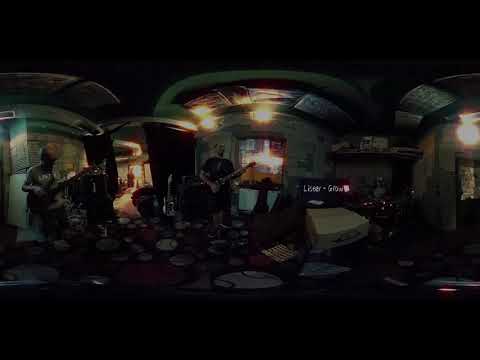This is a dark and distorted panoramic image of a concert in a bar-like setting. The scene features a band on an elevated dais or stage, with two men holding guitars positioned towards the left and center of the image, while a possible drum kit lurks in the shadows, its player obscured. The carpet beneath them is decorated with varying sizes of baseballs. The dim room is illuminated by recessed lighting in the otherwise black ceiling, and a light source on the far right lights up a sign and what appears to be a door. In front of the stage, the view transitions into complete darkness, indicating the audience area is not visible. The image includes thick black borders at the top and bottom, heightening the shadowed, hazy atmosphere.